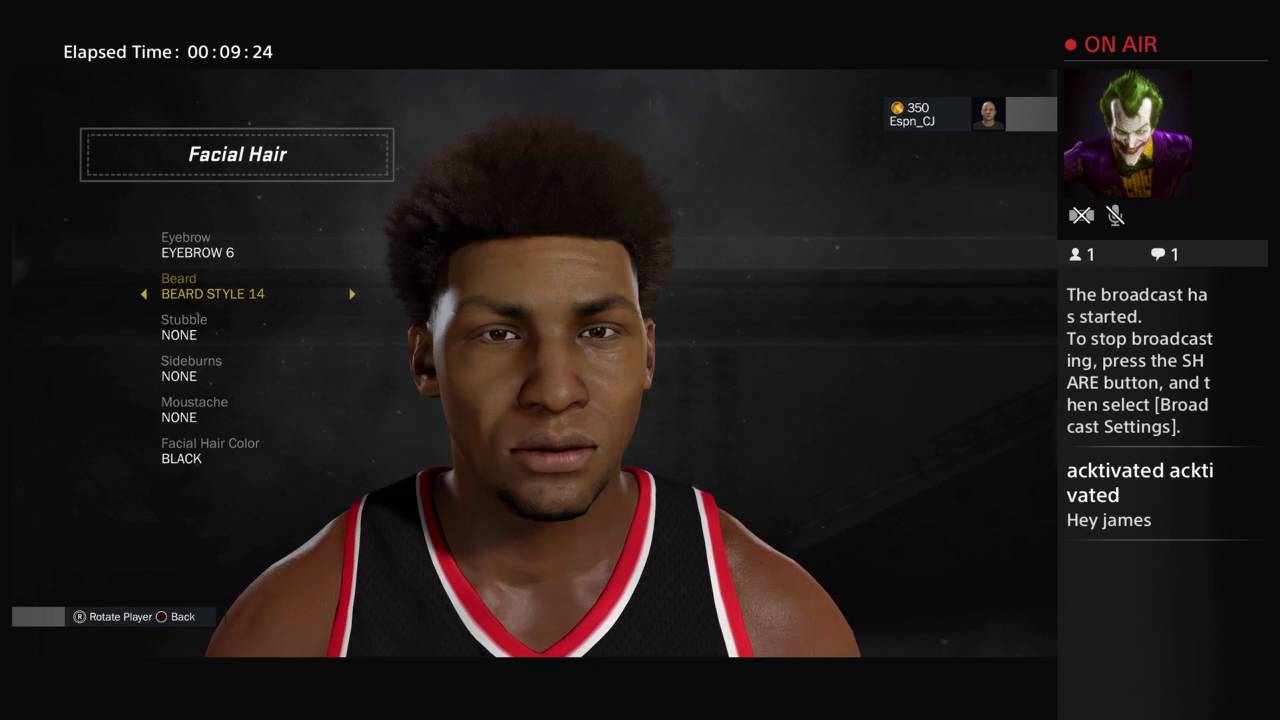**Caption:**

In this detailed screenshot of a PS4 live stream, the streamer is immersed in creating a character on NBA 2K. The main focus of the screen, placed centrally, showcases the intricate character customization features of the game. Sliders and settings for adjusting various aspects of the character's appearance, such as beard style, stubble, sideburns, mustache, and facial hair color, are visible as the player fine-tunes their virtual player's look.

To the right, a separate rectangular section houses the live stream interface. At the top of this section, the "On Air" text accompanied by a small logo signifies that the stream is currently live. Directly below a dividing white line, the streamer's PlayStation icon featuring the Joker is displayed. Further down, crossed-out camera and microphone icons indicate that the streamer does not have their webcam or microphone enabled during this broadcast.

An indicator below these icons shows there is one viewer and one active participant in the chat. The chat box reveals a few messages, including a system notification about how to stop the broadcast and a greeting from a viewer named "activated" saying, "Hey James."

At the top left corner above the NBA 2K window, a timer shows that the stream has been live for 9 minutes and 24 seconds.